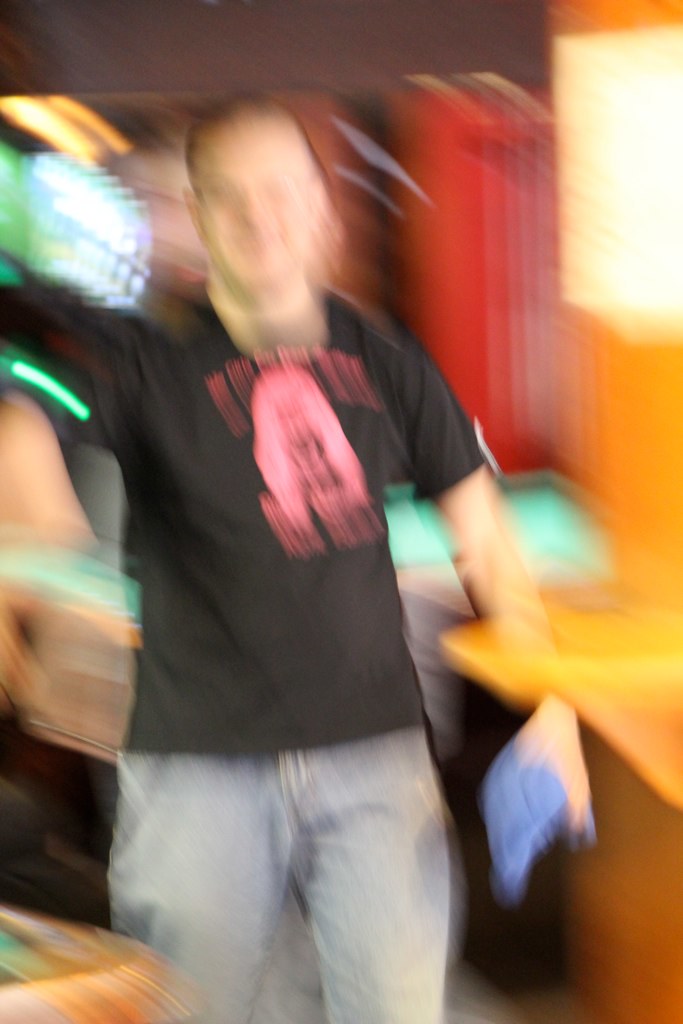This very blurry portrait-mode photograph features a man standing and smiling brightly at the camera, wearing a black short-sleeved t-shirt with some indistinguishable text or imagery that appears in pink, and light denim pants. His face is mostly blurred but a big smile is clearly visible, and he seems to have very short brown hair and possibly glasses. In his left hand, which appears on the right side of the photo as he faces the camera, he is holding something blue—potentially a book, some papers, or a rag—while his right arm is raised. 

He’s situated in what looks like a pool hall, as indicated by the green-felted pool table with wooden sides seen behind him and in the bottom left corner of the photograph. The background is illuminated by bright lights, including some neon that is blurred, and features a bright red section and a small table attached to a brightly lit wall, possibly a window. The context suggests he might have just accomplished something noteworthy while playing pool with friends, adding to the joyful look on his face.